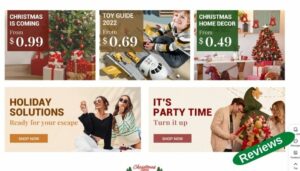This image is an online advertisement layout with a festive Christmas theme comprised of five individual banners. 

1. **Top Left Banner:** This section showcases a beautifully decorated Christmas tree surrounded by red wrapped gifts. A prominent square banner in the image reads, "Christmas is coming from 99 Cents."

2. **Top Middle Banner:** On the right side of the Christmas tree ad, there is an image of a young boy playing with a space toy. Adjacent to the boy, a golden box contains the text, "Toy Guide 2022 from $0.69."

3. **Top Right Banner:** This part of the ad features a small Christmas tree placed on a countertop. To the left of the tree, a green box displays the message, "Christmas home decor from $0.49."

4. **Bottom Left Banner:** This banner depicts two women wearing sunglasses and shopping. The text reads, "Holiday Solutions," with a brown "Shop Now" button displayed prominently.

5. **Bottom Right Banner:** The final banner presents a lively Christmas party scene. The text exclaims, "It's party time. Turn it up," and includes a burgundy "Shop Now" button. A green oblong effect in the lower right corner of this banner contains customer reviews.

These detailed advertisement banners collectively create a vibrant, festive atmosphere tailored for the Christmas season.